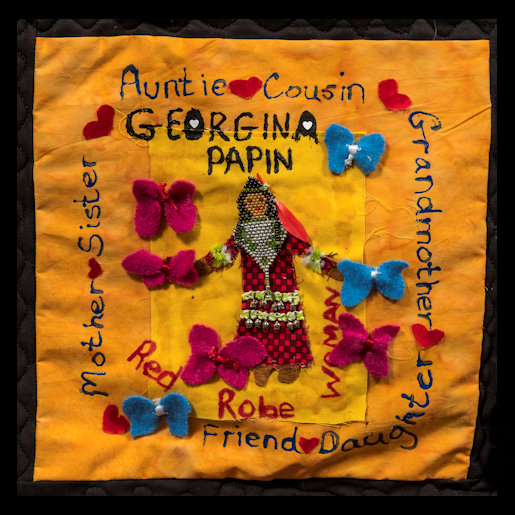The image depicts a handcrafted quilt laid flat on a black surface, bordered by a grayish edge. The quilt's center features a yellow rectangle, while the surrounding fabric is a warm orangish hue. At the heart of the quilt is an intricate depiction of a young Native American woman, created using beads and felt, dressed in a red robe. Surrounding her are felt butterflies—three blue and four purple—adding a whimsical touch.

The quilt is adorned with various words and hearts, indicating familial relationships. Starting from the top and moving clockwise, it reads: "Auntie" with a felt heart beside it, "Cousin" vertically aligned on the right side, "Grandmother" further down, and another felt heart. At the bottom, it says "Friend" and "Daughter", and advancing up the left side, it lists "Mother" and "Sister".

Additionally, the name "Georgina Papine" is inscribed in black, accompanied by the description "Red Robe Woman" at the bottom. This detailed artwork, rich in colors like yellow, red, blue, purple, and orange, appears to be a sentimental creation possibly made by a child or a family member, celebrating their heritage and familial bonds.